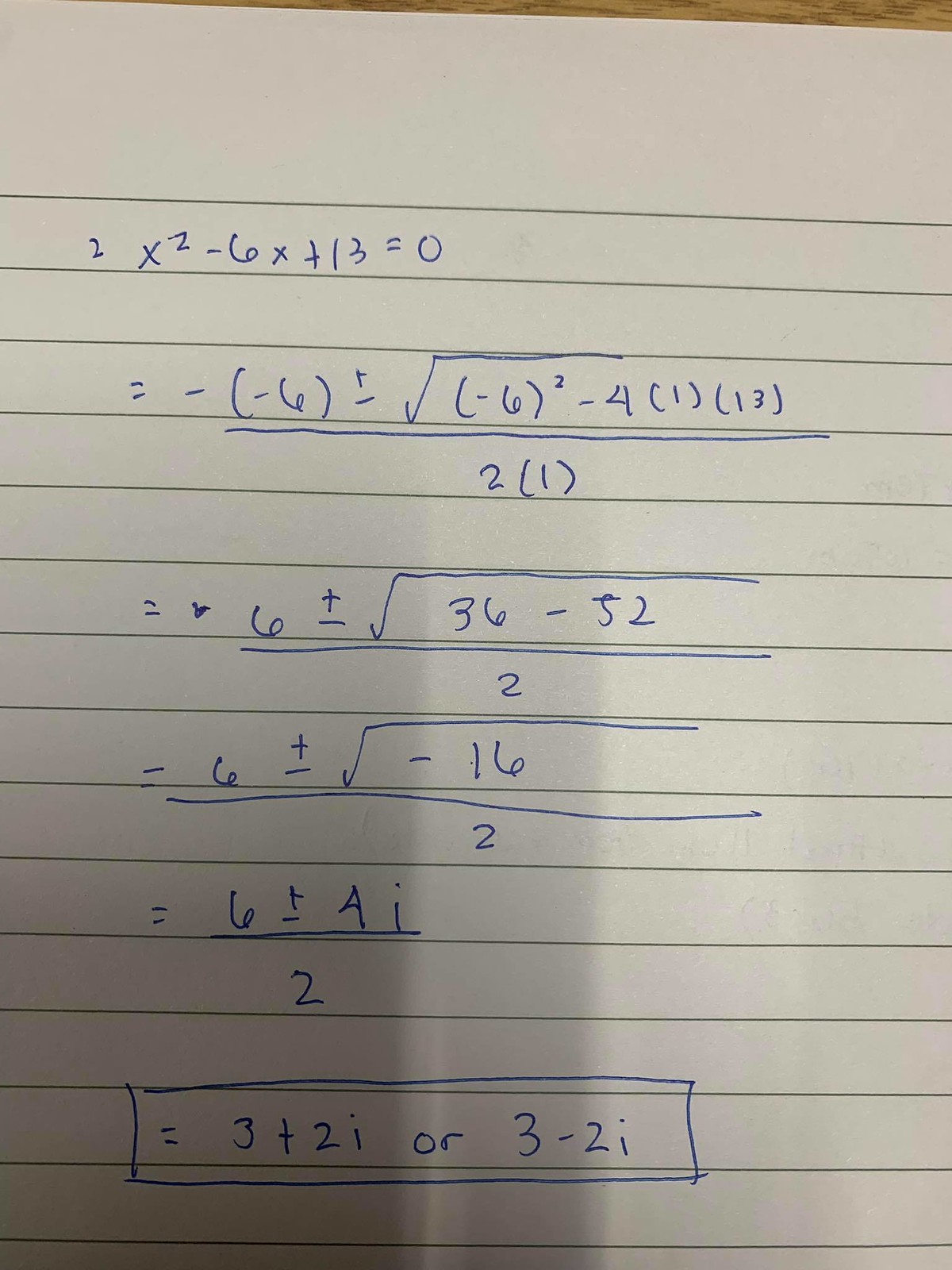The image is a detailed photograph of a sheet of wide-ruled notebook paper with various mathematical calculations written in blue ink, presumably from a ballpoint pen. The heading on the paper features the equation "2x^2 - 6x + 13 = 0," followed underneath by a series of steps utilizing the quadratic formula. Specifically, these steps include expressions such as "-(-6) ± √((-6)^2 - 4 * 1 * 13) / 2 * 1" and several other intermediary calculations leading to the final solutions. The handwriting, albeit somewhat sloppy, remains legible throughout. At the very bottom of the page, the solutions are clearly marked as "x = 3 ± 2i." The notebook paper itself has lines that appear to be a dark or olive-green color. A noticeable shadow spreads across the left side of the paper, creating a contrast with the more brightly lit right side. Additionally, faint, illegible handwriting from the reverse side of the paper can be seen, adding to the layered, lived-in feel of the document.